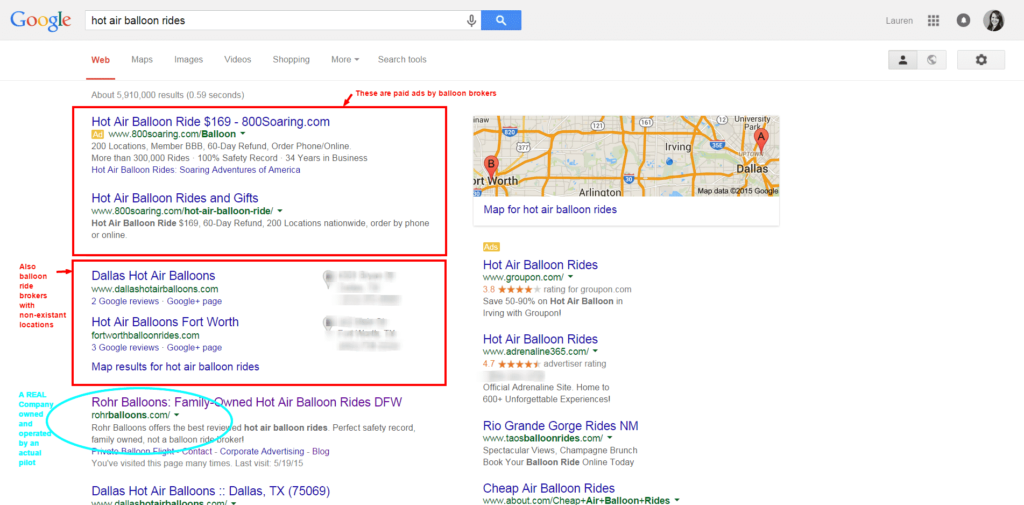A Google search results page for "hot air balloon rides" is displayed. The screen features a traditional Google layout with a predominantly white background and a gray border at the top. The iconic Google logo in its classic colors is situated in the top left corner. At the center, a long white search bar displays the query "hot air balloon rides" in black text. A blue square containing a white search icon is positioned at the end of the search bar.

On the far right side, there's a user profile picture, followed by a sound icon, a vertical ellipsis (three dots arranged in a column), and the name "Lauren" displayed beside them. Beneath the search bar, a navigation menu appears in red text with "web" underlined, accompanied by other options like maps, images, videos, shopping, more, and search tools.

Below the navigation menu, a red notice indicates there are paid ads by balloon brokers. Further down, the screen details the number of search results and the time taken to generate them. The page presents clickable tabs with information on hot air balloon rides, each highlighted by a red border. These tabs link to different sources, with the first tab referencing non-existent locations for balloon rides by brokers. A purple tab labeled "Roar Balloons" is distinguished by a clickable link and a blue circular icon to its left.

On the right side of the screen, a partial map is visible, featuring brown tones with yellow lines representing streets. This map is labeled "map for hot air balloon rides." Below the map, there are links to four additional websites related to hot air balloon rides.